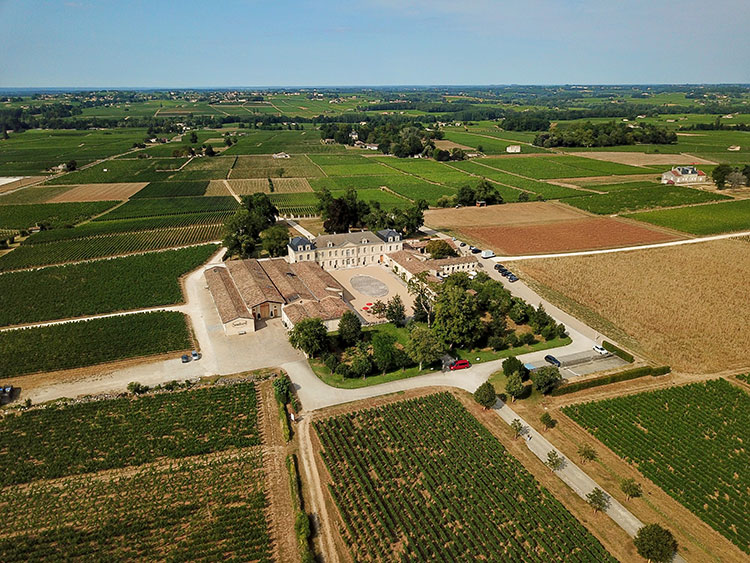This image captures an aerial view of Chateau Sautard, a historic chateau and vineyard set in a vast expanse of farmland. At the center, the main house stands out with its dignified three-story, white-walled structure, capped with a gray roof and blue-roofed wings. Surrounding it is a large paved plaza encircled by several long buildings, possibly stables or outbuildings, with distinct brown roofs. The property is adorned with a lush garden featuring trees and manicured grass in front. Access to the estate appears to be via a tree-lined driveway leading to a grand entrance, complete with a central pool or pond. The entire chateau is surrounded by an organized patchwork of farmland, characterized by different crops showcasing a variety of colors—dark green, light green, beige, and reddish hues. Additionally, clear blue skies frame the idyllic rural setting.